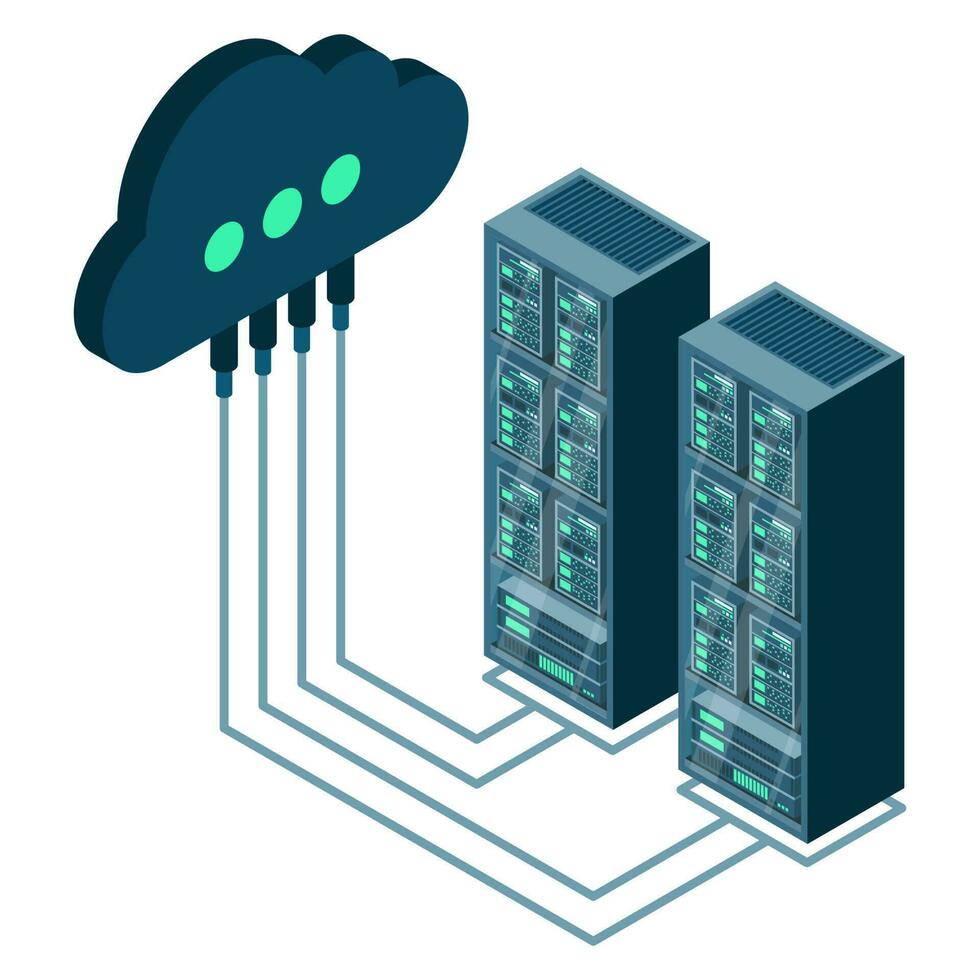This is an isometric digital rendering that visually represents a cloud computing setup. The focus of the image is two substantial server towers, each with six distinct, brightly colored panels that might be indicative of the server's operational status. These servers are equipped with heat vents at the top, emphasizing their function in a data center-like environment. Light blue lines, symbolizing electrical or data connections, originate from these servers and extend outwards. These lines converge on the left side of the image, transitioning vertically before connecting to a prominent 3D blue cloud. This cloud features three green power indicators arranged horizontally, signifying active connectivity. Cylindrically shaped connectors, matching the dark blue color of the cloud, taper into lighter blue lines that seamlessly integrate into the holes at the base of the cloud. Predominantly, the image employs various shades of blue to highlight the technological elements, with touches of green and aquamarine to illustrate operational signals and electronic interfaces.